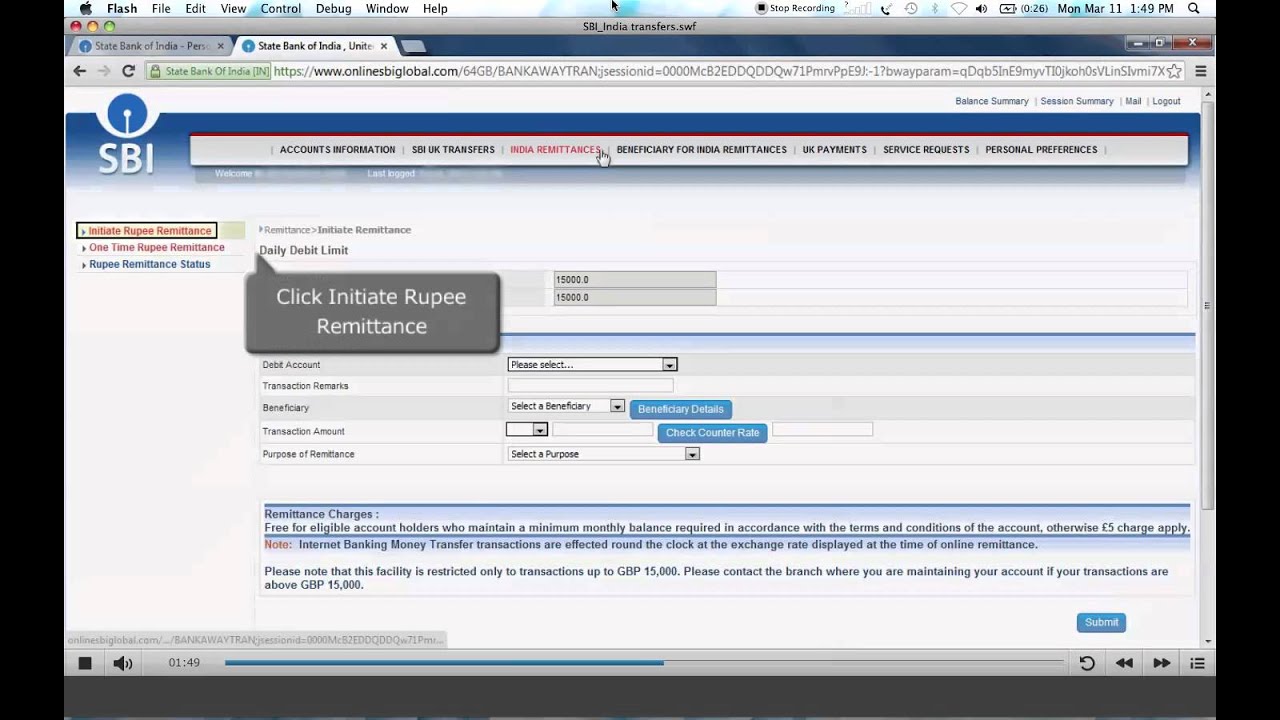This image is a screenshot from the 'India Transfers' application, displaying its detailed user interface. The layout features vertical black rectangles on both the far left and far right borders, extending from top to bottom. At the very top of the screen, there is a light blue horizontal band with black text, detailing a menu bar that reads: "Apple," "Flash," "File," "Edit," "View," "Control," "Debug," "Window," and "Help." 

Adjacent to this menu bar, to the right, are several icons: a square inside a circle, a "Stop Recording" button, a phone icon, a directional arrow within a circle, Bluetooth icon, Wi-Fi signal indicator, speaker icon, battery level indicator (reading 0.26 in parentheses), and the date and time displayed as "Monday, March 11th, 1:49 PM." This section concludes with a magnifying glass icon.

Beneath the menu bar, two browser tabs are open, both labeled "State Bank of India." Below the tab titles, the screen features a prominent "SBI" logo in white text on the left, followed by a long white rectangle with a thin red line at its top edge, spanning from left to right. This section includes the following menu options in black text: "Accounts Information," "SBI UK Transfers," "India Remittances" (in red text), "Beneficiary for India Remittances," "UK Payments," "Service Requests," and "Personal Preferences."

Further down the interface, on the left side in red text, it says "Initiate Rupee Remittance," followed by a secondary option, "One Time Rupee Remittance," and in black text, "Rupee Remittance Status." To the right of these options, there is a mention of the "Daily Debt Limit" and a clickable instruction to "click Initiate Rupee Remittance." 

The lower portion of the screen contains various fields labeled "Debit Account," "Transaction Remarks," "Beneficiary," "Transaction Amount," and "Purpose of Remittance." At the very bottom, there is a blue rectangle featuring a "Submit" button in white text, intended for finalizing the transaction.